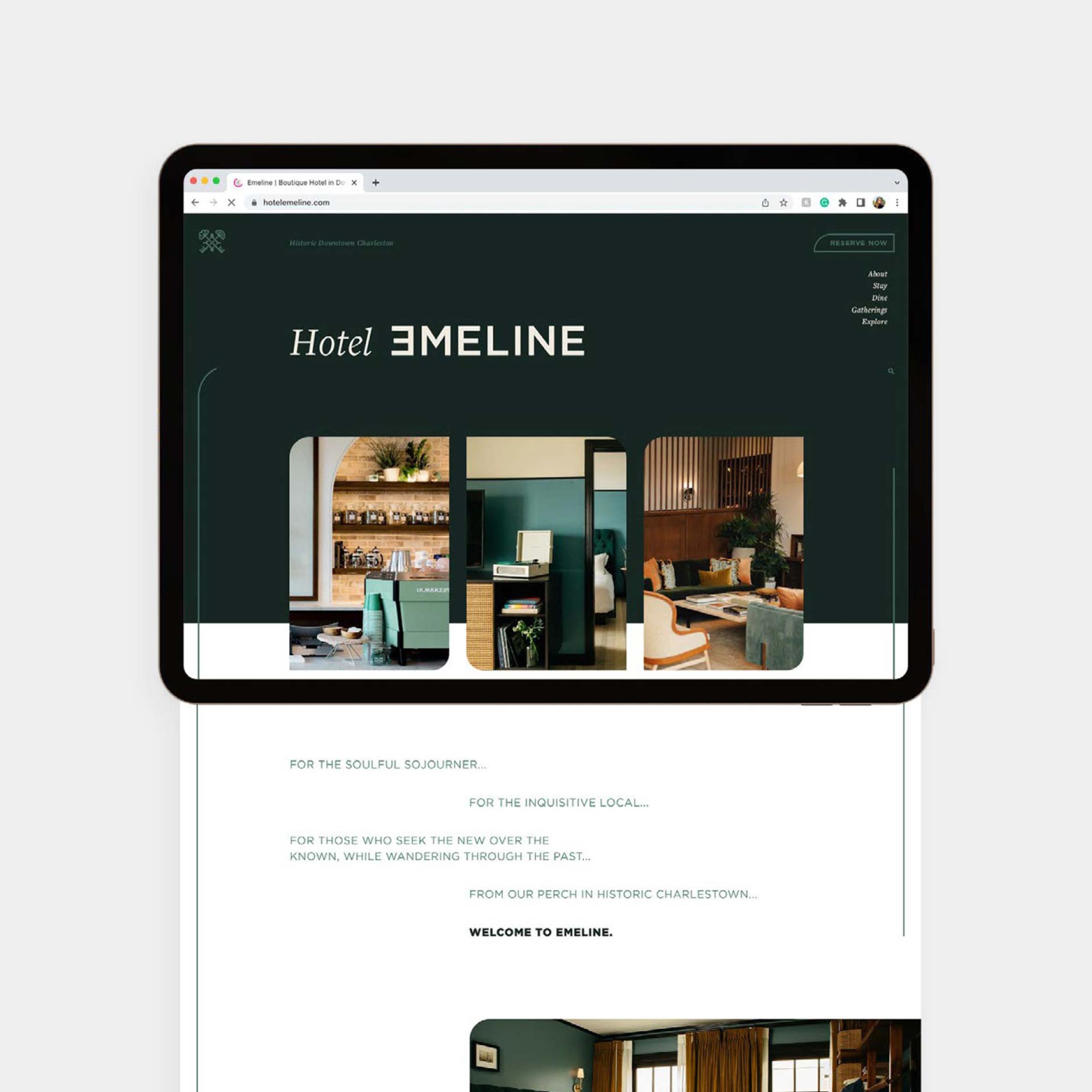The image features a serene gray background with an iPad displaying the interior of Hotel Emmeline. Notably, the hotel name includes a distinctly styled backwards 'E' for the first letter. The iPad screen itself shows a website with the hotel's address, a tab bar, and a profile picture. The page prominently displays a welcoming message specifically designed for various types of guests: "for the soulful sojourners," "for the inquisitive local," and "for those who seek the new overtime, known while wandering through the past." The message concludes with a warm greeting from "our perch in historic Charleston," inviting viewers to Hotel Emmeline. The image also includes the top portion of the hotel building, framed by two elegant, floor-length curtains.